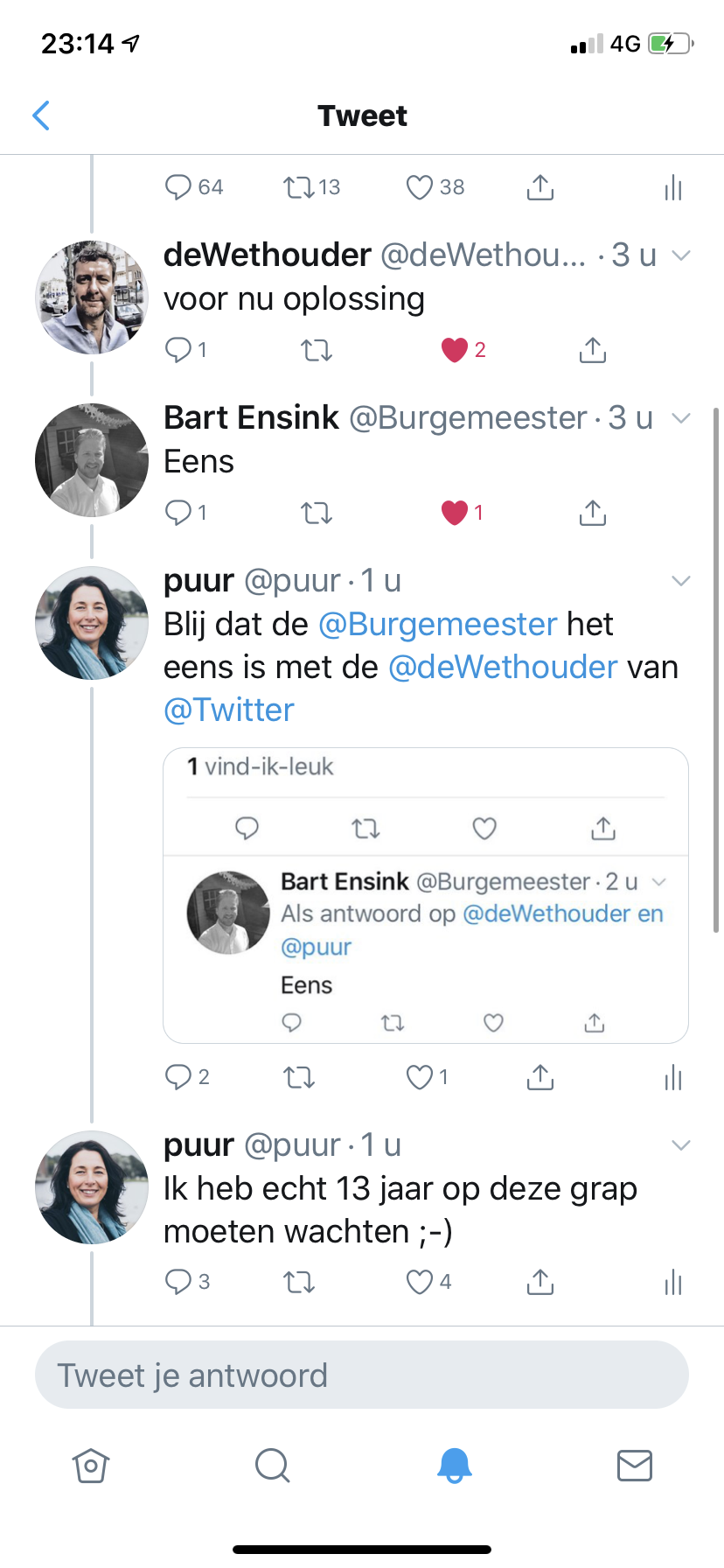This image is a detailed screenshot taken from the Twitter app on an iPhone. The entire frame of the image is occupied by the screenshot itself. At the very top, the time is displayed as 23:14 on the left, while on the right, there are signal bars, a 4G indicator, and a battery icon with a thunderbolt symbol and a green filling. Centrally positioned at the top is the word "Tweet" in black text. The main background of the screenshot is predominantly white. 

In the center, we see various interactive elements associated with a tweet, including text boxes and icons for likes, retweets, and replies, each accompanied by numbers: 64 for replies, 13 for retweets, and 38 for likes, represented by a text box, arrows, and a heart, respectively. Notably, there are thumbnails to the left side of the tweets, each circular and showing the profile pictures of the users – a woman and two men. The usernames visible beside the thumbnails include Dewithoder, Bart Ensink, and P-U-U-R. 

Further down, the conversation continues, though the text is in a different language and thus not easily interpretable. Red hearts, indicating likes, punctuate the dialogue. Along the bottom of the interface, there's a navigation bar displaying icons: a house, a magnifying glass, a bell – colored in blue, and an envelope. The overall setting strongly suggests that this is a snapshot of a Twitter exchange on an iOS device, with common UI elements distinctly visible.